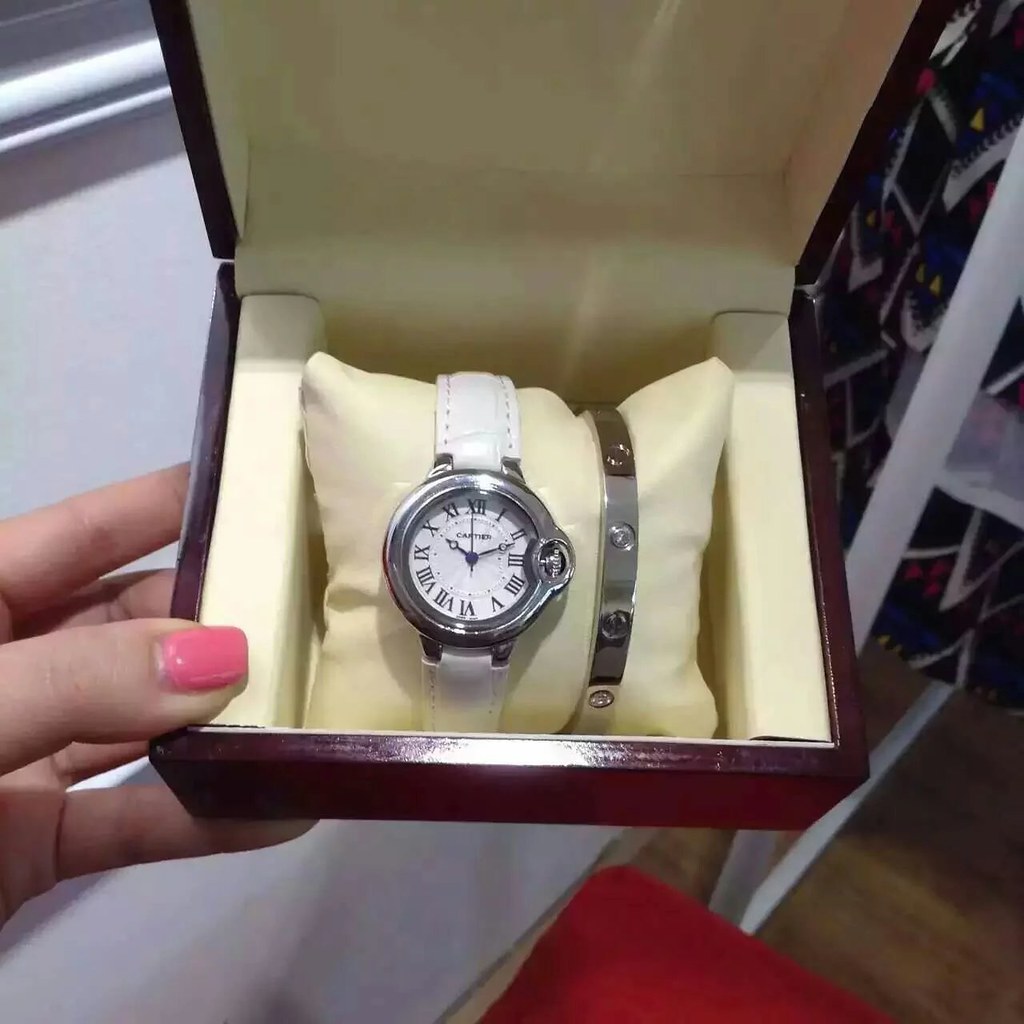The image features an elegant wristwatch with a pristine white leather band, showcased against a richly textured brown case that appears to be made of wood. The watch displays classical Roman numerals on its face, with the brand name faintly discernible as "CA," partially obscured by the second hand positioned slightly past the 2 o'clock mark. The small hand is pointing towards the numeral 10. The luxurious case cradles the watch on a soft, white cushion, enhancing the sense of opulence. Adjacent to the watch is what seems to be a bracelet, adding an additional touch of sophistication. The watch and its accessories are being held aloft by a person whose thumb, adorned with pink fingernail polish, is visible in the shot.